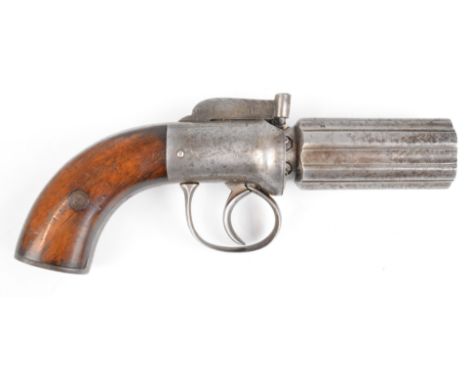This image features a vintage pistol with a distinctly old-fashioned appearance, likely handmade and not commonly seen today. The gun boasts a curved wooden grip, riveted together at its center, showcasing a glossy but worn brown finish with varying degrees of polish throughout. The wooden handle is accented by a silver metal border. The trigger and the finger guard, which are also made of silvery metal, display some dullness typical of an aged weapon. Attached to the handle is a brown tube, adding to the antiquated charm of the gun. The side-mounted cocking mechanism further emphasizes its unique craftsmanship. The barrel resembles a revolver's, featuring indentations that suggest multiple chambers, though their exact count is obscured by wear. Set against a stark white background, this pistol stands as a focal point, invoking a sense of historical intrigue.